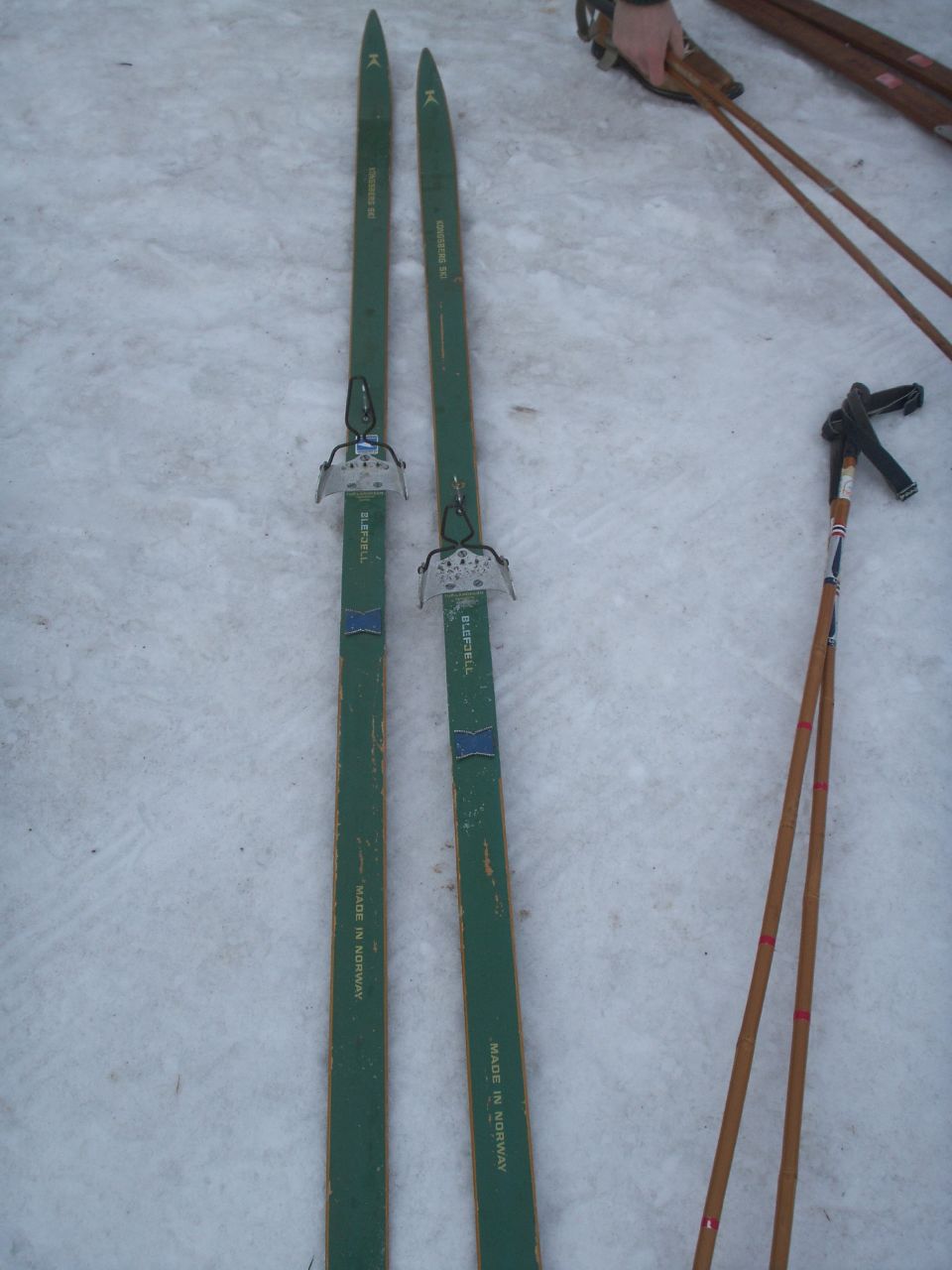The image is a detailed photograph taken from a standing level looking down onto icy, packed-down snow. In the scene, a pair of green cross-country skis, long and sword-like with pointy ends, lay on the snow. The skis feature silver harnesses with black, clamp-like attachments, showing signs of wear with some green paint scratched off. Accompanying the skis are two sets of wooden-colored ski poles with black handles, one of which is held by a person in the upper right corner, suggesting they are preparing to ski. In the background, there is a hint of another set of wooden-toned skis. The entire setup rests on a white, snowy surface, giving a sense of a ready-to-go skiing adventure.